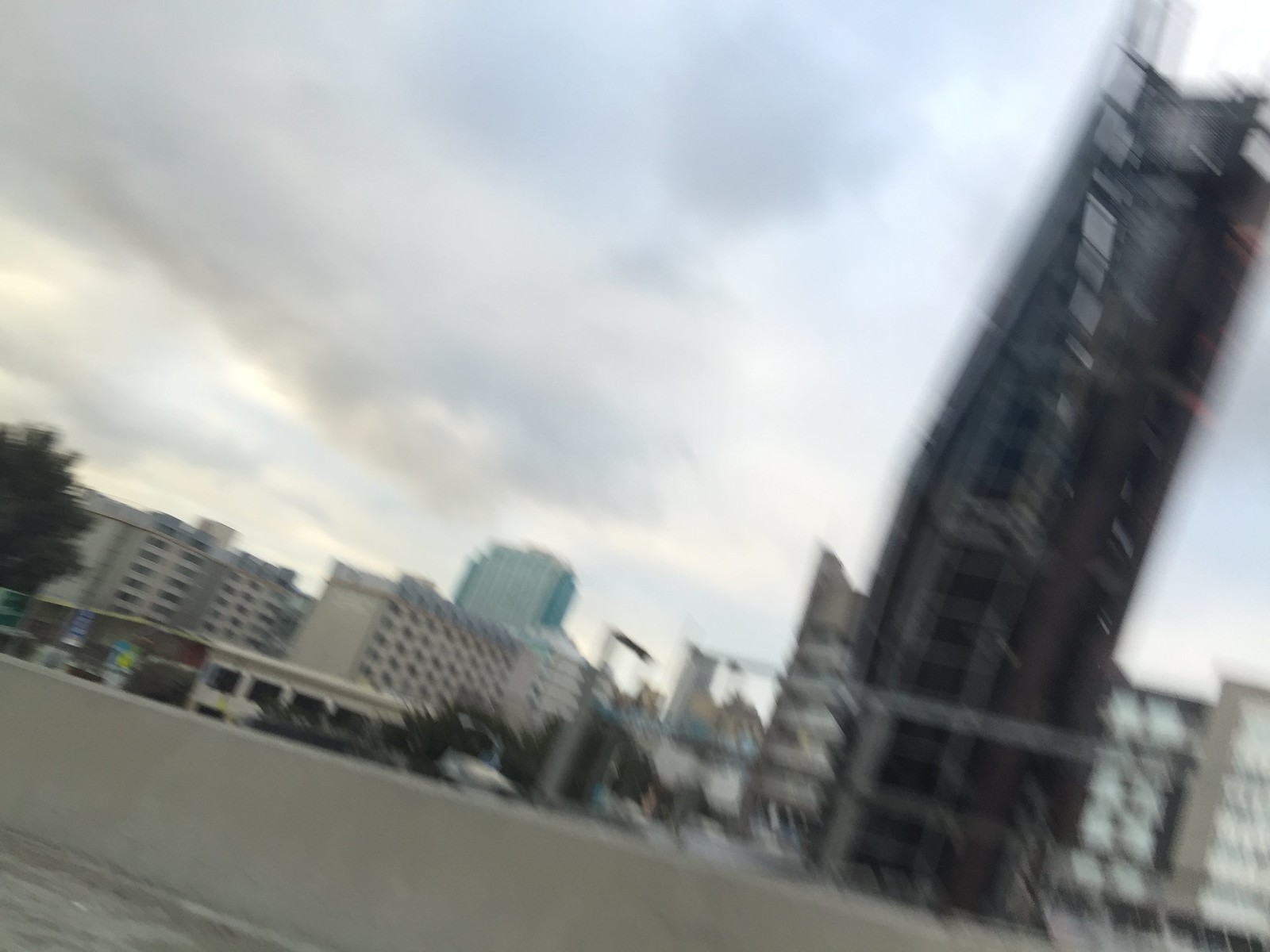A blurred photograph captures an urban landscape from the vantage point of what appears to be the top of a parking garage. A towering black skyscraper with indistinct white sections dominates the right side of the image. A waist-high, gray or white cement wall runs along the bottom edge, hinting at the parking garage setting. The cityscape unfolds in the background, featuring a mix of white apartment buildings and a prominent blue structure in the far distance. A solitary tree is visible to the left, while the sky above is overcast, casting a muted light over the scene. The absence of people or text adds to the sense of motion and disorientation in this blurred, out-of-focus urban snapshot.